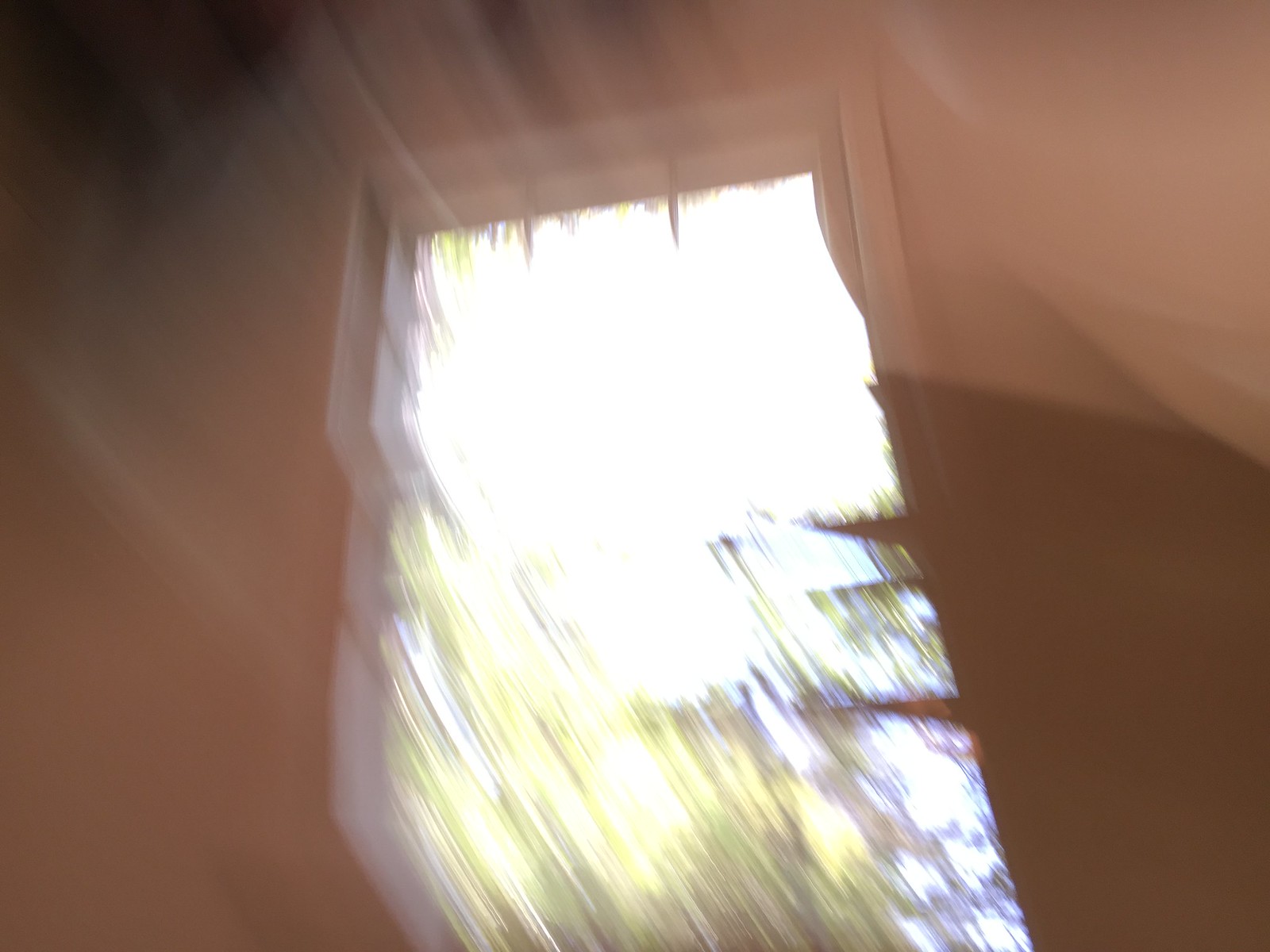The image depicts a highly blurred scene, making it challenging to discern precise details. However, it appears to capture an exterior wall of a building from the inside. The wall, which seems to be a reddish-brown color, features an opening that resembles a window or doorway. The main light source emanates from this opening, illuminating the space with daylight. Outside the window, the bright sky and some tree leaves are visible, suggesting a natural setting. The window itself is framed by a white border and windowsill. Due to the poor lighting and significant blur, further details are indiscernible.